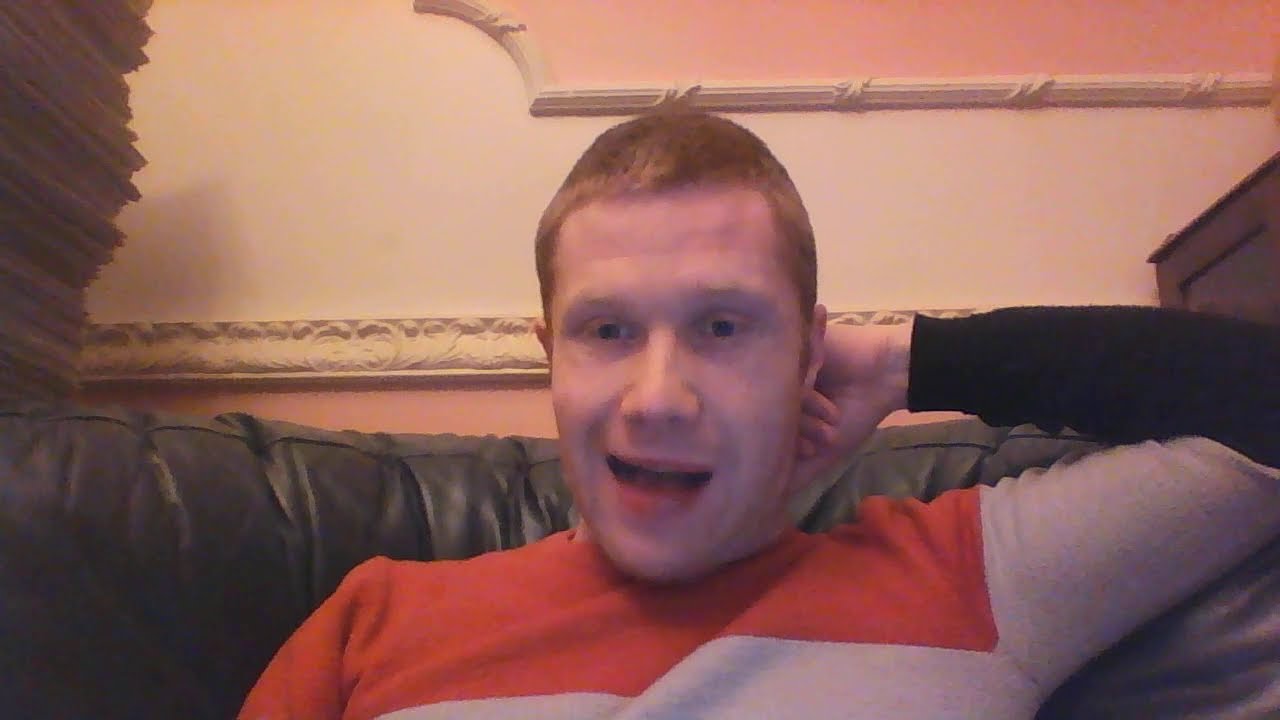This screenshot captures a young white male, likely in his early 20s, with reddish-brown hair and blue eyes, sitting on what appears to be a black leather sofa. He is engaged in a video chat, looking directly at the camera with a slight smile and his mouth slightly open, mid-sentence. His left arm is raised, scratching the back of his head. He is dressed in a distinctive long-sleeve sweater that features a variety of block stripes in colors like brown, red, black, orange, and gray. The background reveals a pink wall adorned with intricate decorative designs and a white molding running across it. Flanking the sofa are pieces of brown furniture; to the left, there is a stack of newspapers, while to the right, there is a cabinet or shelf. The image quality is somewhat grainy and pixelated, suggesting the video quality wasn't optimal during the capture.